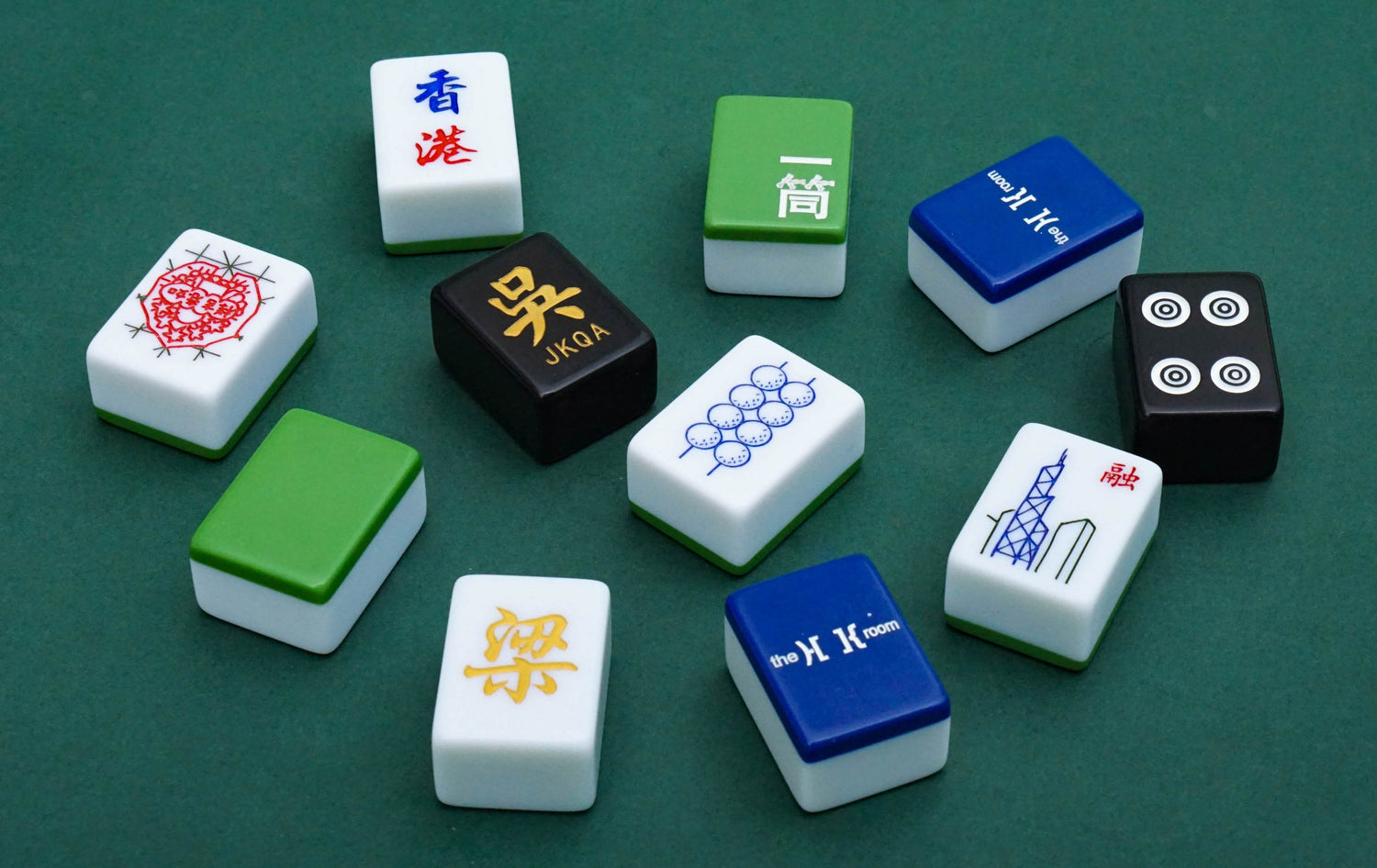This photograph captures a well-lit arrangement of 11 Mahjong tiles on a dark green background, possibly a tablecloth. The tiles are organized in a loose circular pattern with two tiles placed centrally. The colors of the tiles include five white, two green, two black, and two blue. The tiles are uniform in size and material, each displaying unique designs and markings, except for one solid green tile.

Among the tiles, the white ones bear the most traditional Mahjong images, including intricate designs, bullseye-type circles, Chinese characters, and other detailed patterns. Two white tiles feature rows of blue circles with lines through them, and another white tile depicts skyscrapers in blue and black alongside a red Chinese character. Additionally, one white tile has a green cover with white details, and another is partially white with a dark blue top inscribed with small, unreadable words.

The two black tiles are prominent: one has a gold Chinese symbol with the letters "JKQA" beneath it, positioned centrally, while the other showcases four bullet target designs arranged in pairs. The blue tiles are similarly intriguing; inscribed in white on one is the phrase "the HK room," though the small wording on the other remains unreadable.

Overall, the detailed Mahjong tiles, arranged in a semi-circle with two central pieces, display an array of colors and intricate designs against a rich green background, catching the eye with their varied imagery and unique characteristics.